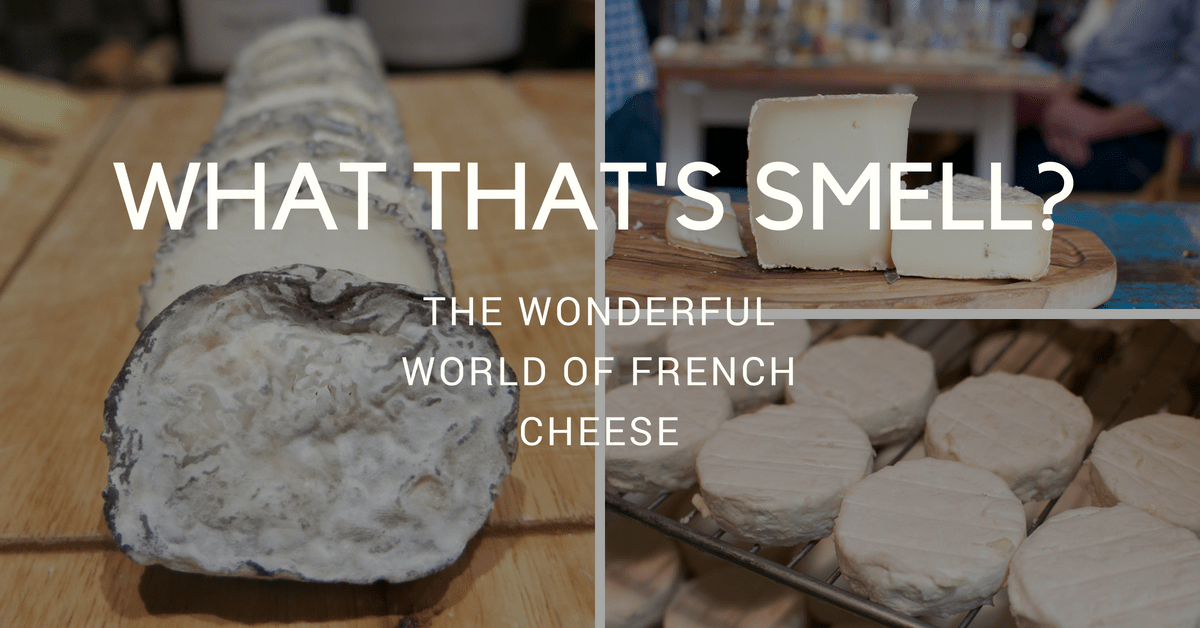This image is a composite of three photographs, each showcasing different types of French cheese, with superimposed text in a minimalist sans-serif white font. The main text at the center reads, "WHAT'S THAT SMELL?" in all caps, with a smaller, thinner caption below stating, "The wonderful world of French cheese." The layout is landscape-oriented, with the left side featuring a tall portrait photo of a log-like cheese sliced into flattened, round-edged rectangles, resting on a light wood surface. The two right-side photos are stacked: the top image depicts several wedges of white cheese standing upright on a wooden platter, with indistinct figures sitting at a table in the background; the bottom image shows round discs of white cheese arranged on a cooling rack, with more similar discs visible below. The overall scene is set indoors and emphasizes the varied textures and forms of French cheese, captured with a realistic photographic style and separated by light gray dividers. The color palette includes shades of white, off-white, tan, beige, black, brown, blue, and teal, blending warmth and contrast to highlight the delectable details of the cheeses.